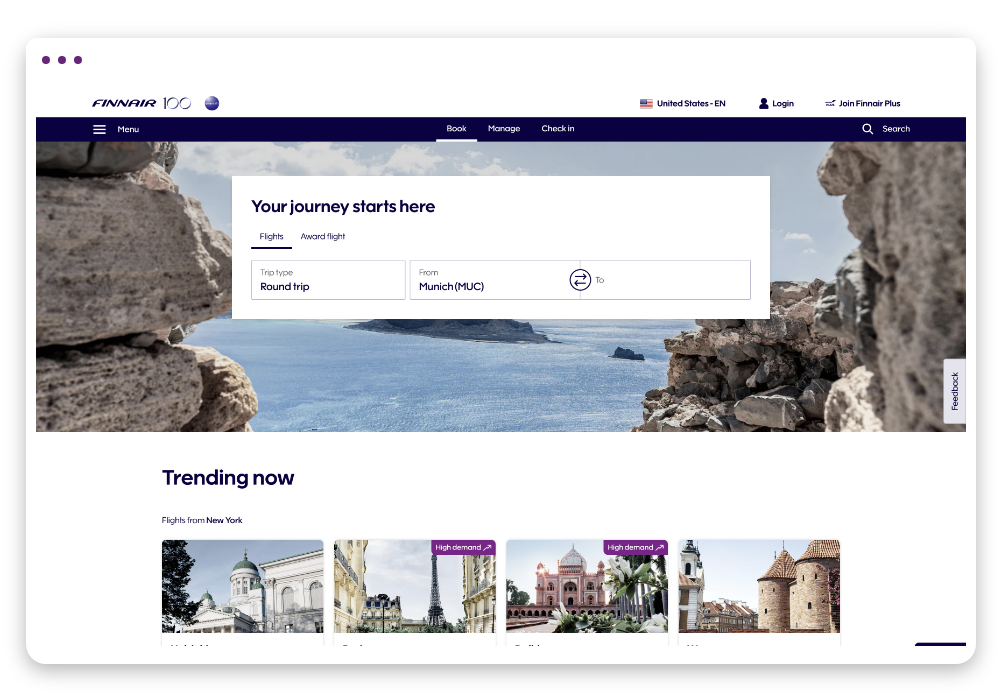The image depicts a Finnair web page featuring a predominantly white background. At the very top, a dark navy blue strip runs horizontally, containing options labeled "Menu," "Book," "Manage," "Check-in," and "Search," all aligned from left to right. Above this strip, still set against the white background, the text "United States - EN" is displayed next to an American flag icon, indicating language and region settings. There is also an icon of a human silhouette with the option to "Log in" and another text stating "John Finnair Plus" indicating user account information. 

In the upper left-hand corner, three horizontal purplish dots are shown, likely representing a menu or additional options. Below this, a high-resolution image captures a stunning scene, presenting a vast, watery expanse interrupted by a central island, framed by rocky outcrops on both the left and right sides. The photo, taken from an elevated vantage point, also showcases a vibrant sky adorned with white, fluffy clouds. 

Overlaying this picturesque landscape, bold text reads "Your journey starts here," inspiring users to embark on their travels. Below this prompt are options such as "Flights," "Award Flight," "Round Trip," and "Trending Now," each likely accompanied by corresponding images, inviting users to explore various booking choices and travel inspiration.